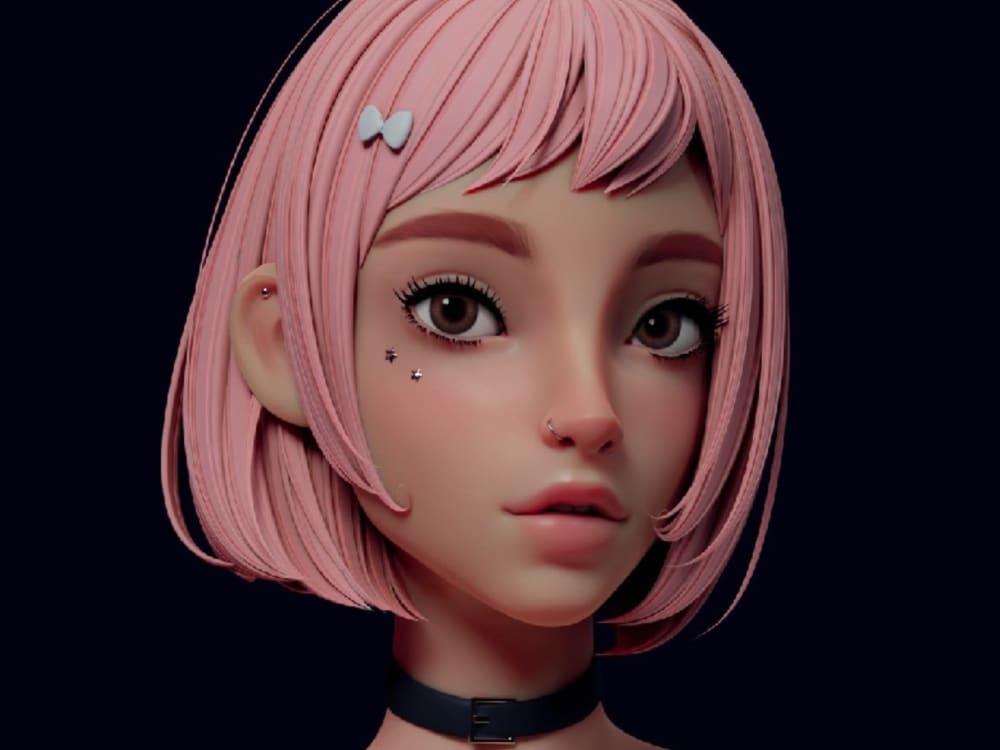In this computer-generated image set against a completely black backdrop, a Caucasian woman gazes directly into the camera with wide, expressive brown eyes. Her full, pinkish lips and light brown eyebrows add to her captivating appearance. She sports a nostril piercing and has two small star tattoos adorning her upper left cheek. One ear, visible through her short, pink hair, features a piercing at the top. Her hair, which falls just halfway down her neck, is accentuated by a small white bow on the left side. Around her neck, she wears a black collar that is centrally positioned at the bottom of the image, completing her distinctive look.